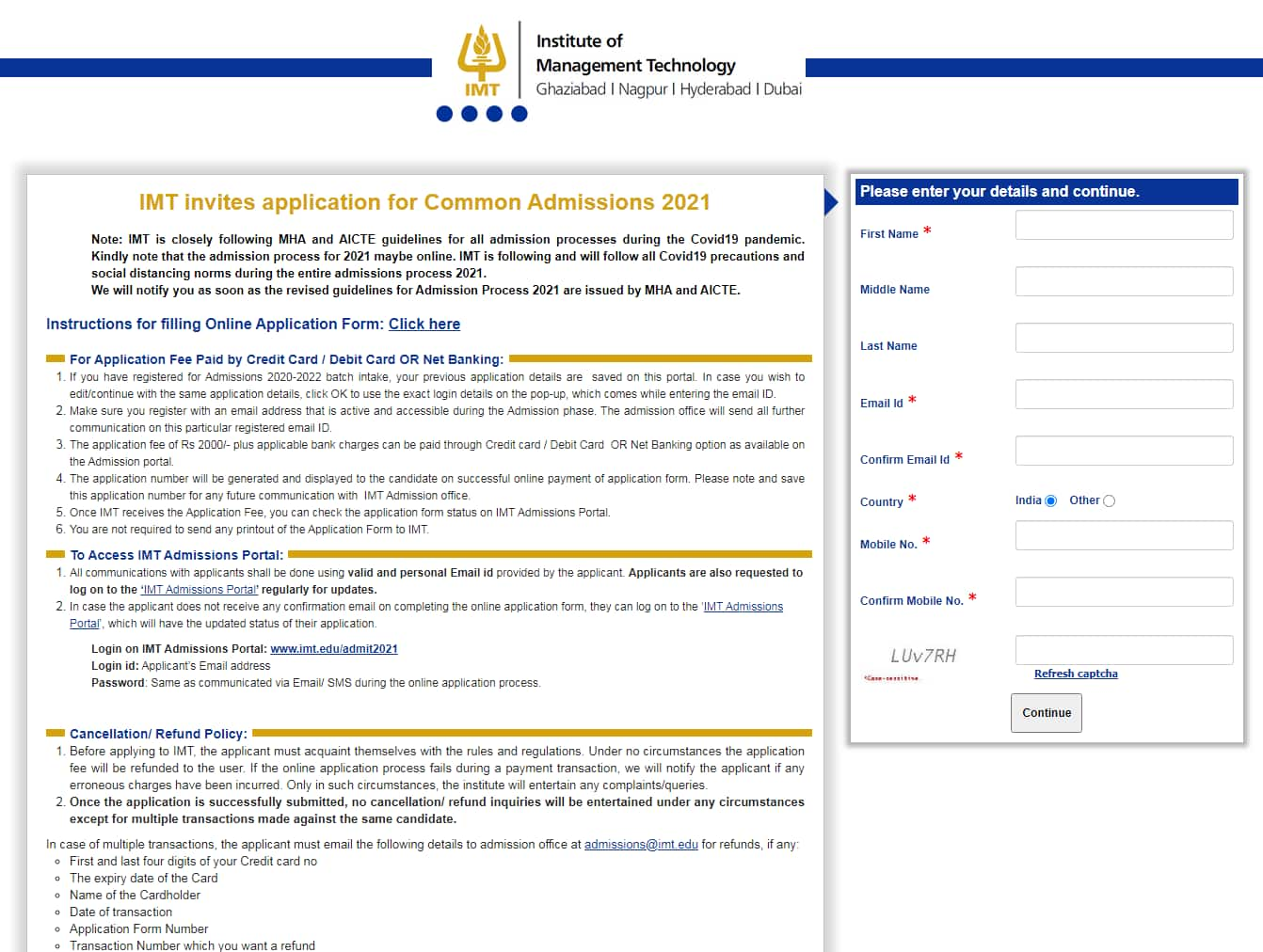The website for the Institute of Management Technology (IMT) prominently displays "IMT" in a gold logo at the uppermost part, framed by navy blue bars on the left and right sides. Beneath the IMT logo, there are four dots lined up horizontally. The primary headline invites applications for the Common Admissions 2021. An instructional note is situated at the top, followed by a clickable "Instructions for Filling Online Application Form" link in blue. 

The next section provides information on the application fee, which can be paid via credit card, debit card, or net banking. Below this is a gold line divider. 

Further down, there is a section dedicated to accessing the IMT admissions portal, accented with another gold bar. The cancellation and refund policy is detailed at the bottom, accompanied by a similar gold bar. Each section includes fine print that directs applicants on the steps for applying, payment methods, and resolving issues with multiple transactions, with specific instructions detailed in black at the very bottom.